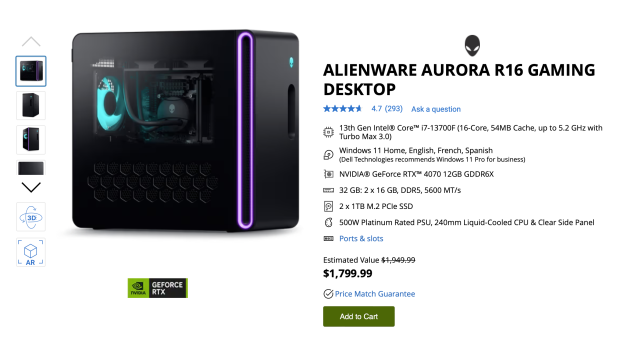**Product Page for Alienware Aurora R16 Gaming Desktop Computer**

On this detailed product page, the Alienware Aurora R16 gaming desktop computer is showcased prominently. The left side of the page features a column with small clickable icons, allowing users to view larger images of the computer. The main section displays a high-resolution image of the desktop computer. 

The computer's casing is sleek and black with a semi-transparent panel on the side, revealing internally illuminated blue components. A clearly visible fan is among these components. The exterior is adorned with a fluorescent purple strip and a glowing blue Alienware icon, enhancing its futuristic aesthetic. 

Beneath the image, a disclaimer mentions "GeForce RTX Samsung," likely indicating a key feature related to the computer's graphics capabilities. On the right side, a text description offers more details about this high-performance gaming machine.

The Alienware Aurora R16 is introduced with the logo of Alienware, a black alien skull. It has an impressive rating of 4.7 stars based on 293 reviews. A hyperlink invites users to "Ask a Question."

The detailed product description highlights its robust specifications:
- 13th Gen Intel Core i7-13700F, 16-Core, 54MB Cache, with speeds up to 5.2GHz using Turbo Max 3.0.
- Windows 11 Home operating system (available in English, French, and Spanish). Dell Technologies recommends Windows 11 Pro for business use.
- NVIDIA GeForce RTX 4070 graphics card with 12GB GDDR5X memory.
- 32GB of RAM (2x16GB GDDR5, 5600MT/s).
- Dual 1TB M.2 PCIe SSD storage.
- 500W Platinum-rated power supply unit (PSU).
- 240mm liquid-cooled CPU.
- Clear side panel showcasing internal ports and slots.

An estimated value is shown at $1949.99, which is slashed out to indicate a discount. The current price is displayed as $1799.99. Additional features include a "Price Match Guarantee" and an "Add to Cart" button in green with white text overlay.

This comprehensive product page effectively presents the Alienware Aurora R16, catering to gaming enthusiasts with its high-end specs and visually appealing design.